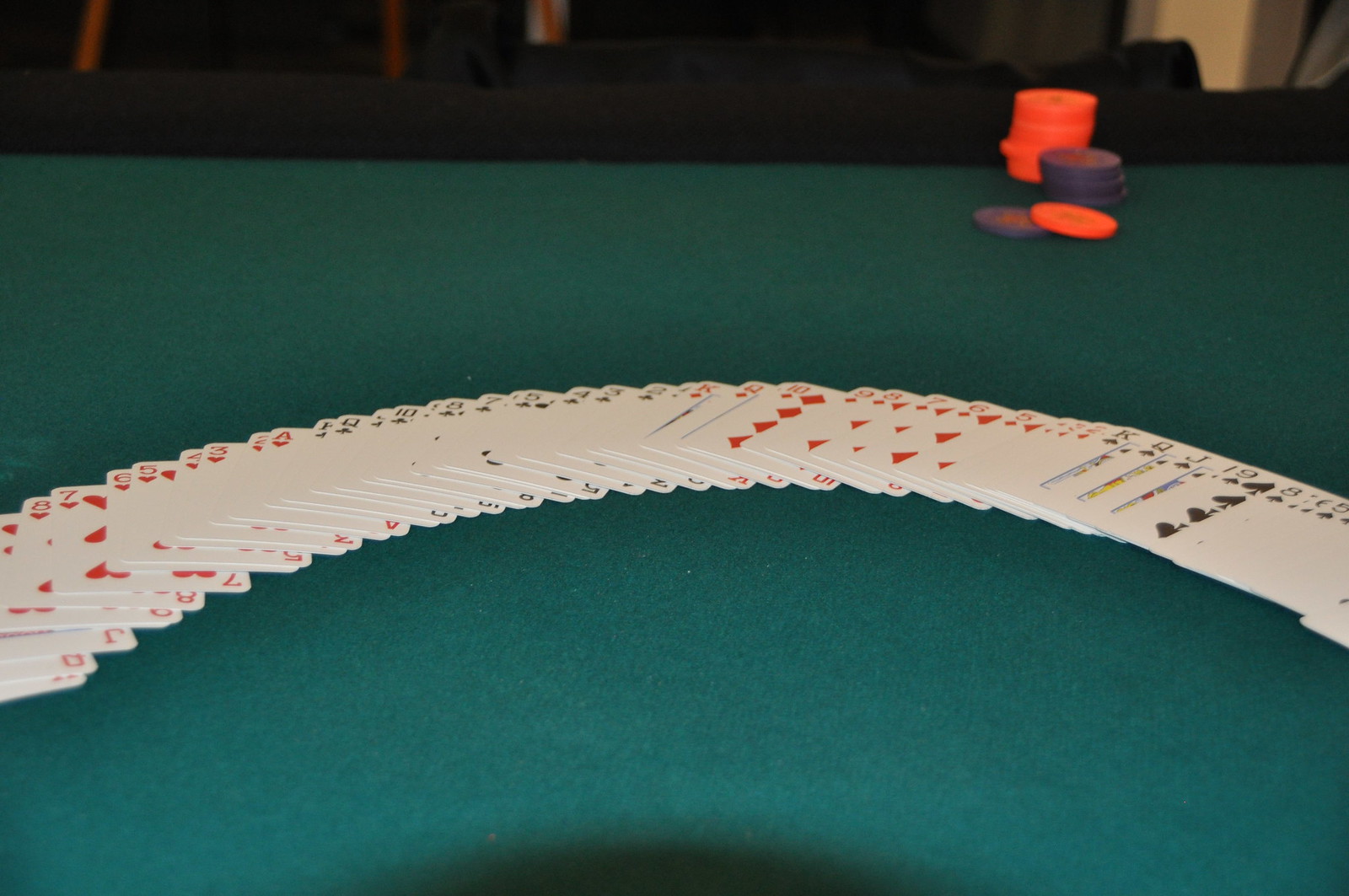A slightly out-of-focus color photograph captures a dealer's table at a casino, predominantly enveloped by an expanse of greenish-blue felt. Spanning across the table from left to right is a deck of playing cards meticulously fanned out in a shallow arc. Upon close inspection, it becomes apparent that the cards are arranged in perfect sequential order. Visible among the array are hearts starting from the ace through to the eight, followed by clubs with visible king and queen cards, then diamonds, and finally spades taking up the rightmost section.

Dominating the bottom portion of the image is a pronounced arc-shaped shadow, possibly cast by the dealer's head, adding a subtle element of human presence. On the right side of the table, a neatly organized stack of poker chips is visible. These chips are colored orange and blue, featuring a tall stack of orange chips next to a shorter blue stack, with an additional single blue chip and single orange chip slightly overlapping each other.

Towards the top of the image, although blurred and barely visible, are hints of chairs or other pieces of furniture, giving a sense of the casino's bustling environment beyond the table.